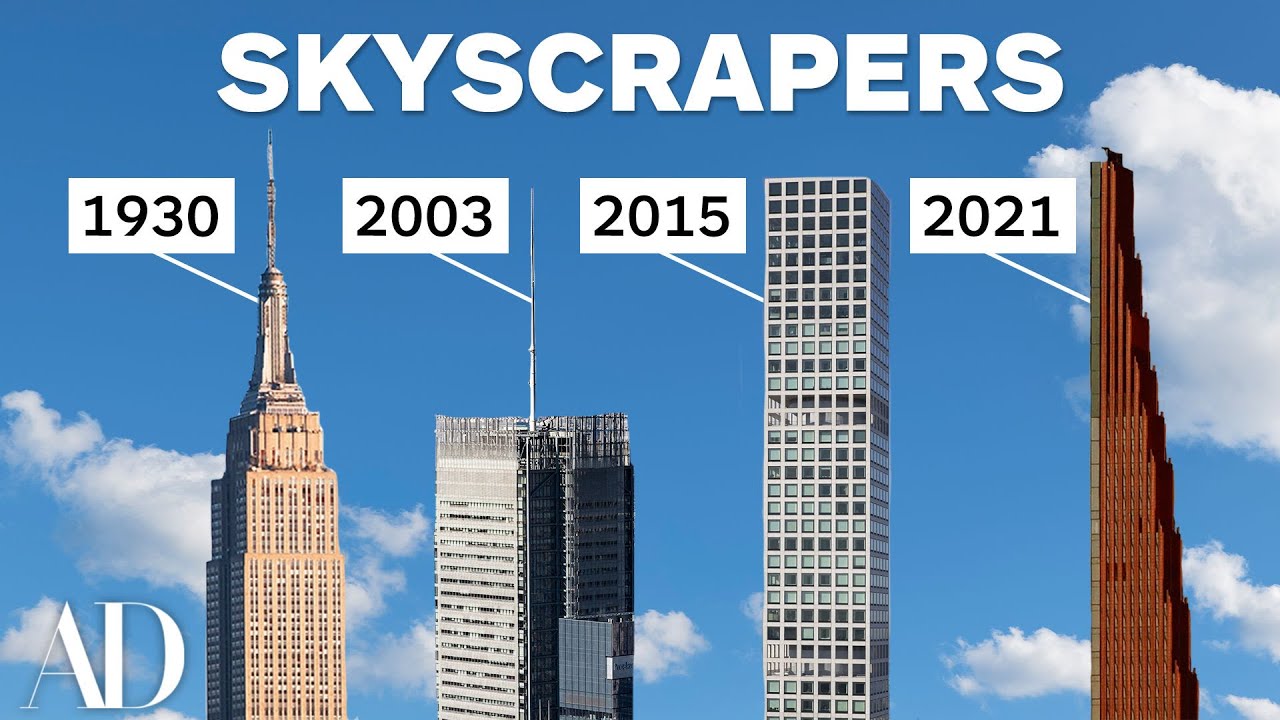The image features a detailed digital rendering of various skyscrapers set against a blue sky adorned with white, fluffy clouds. At the top of the image, bold white letters spell out "SKYSCRAPERS." From left to right, the image showcases four skyscrapers, each labeled with corresponding years in white boxes: 

1. A brown building with a skinny top marked "1930s."
2. A gray building featuring an antenna on top marked "2003."
3. A much taller, rectangular building from "2015."
4. A uniquely shaped building that is thicker at the bottom and thinner at the top, labeled "2021."

Additionally, the bottom left corner of the image prominently displays the letters "AD" in big, bold white text.